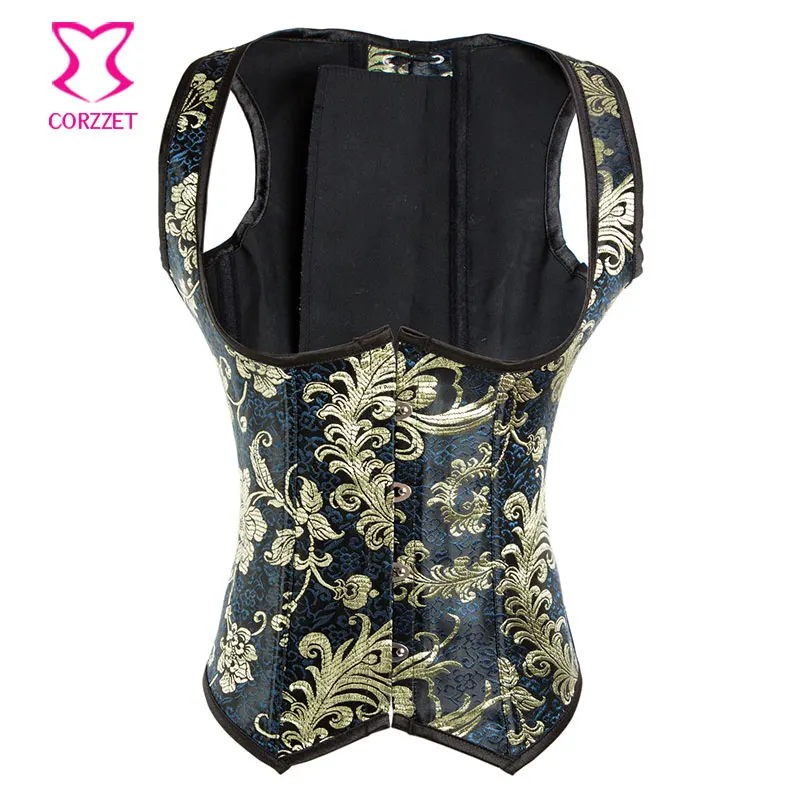This detailed image depicts a vintage-style corset, advertised as women’s clothing, with a blend of historical flair. In the upper left corner, there is a hot pink cartoon outline of a corset labeled "C-O-R-Z-E-T" in bold letters, presumed to be the brand's trademark. The corset features an antique design with a striking teal blue-black base adorned with a white fern and floral pattern along the front and back. Gold leafing adds an elegant touch to the floral motifs. The garment has four distinctive golden buttons down the center for closure, which gives it a timeless, Renaissance-era appeal. From a back view, the interior lining of the corset is purely black, and unique jagged edges at the bottom front, resembling vampire teeth, add to its unique aesthetic. This corset includes large armholes and a generously sized head opening, designed to fit comfortably.